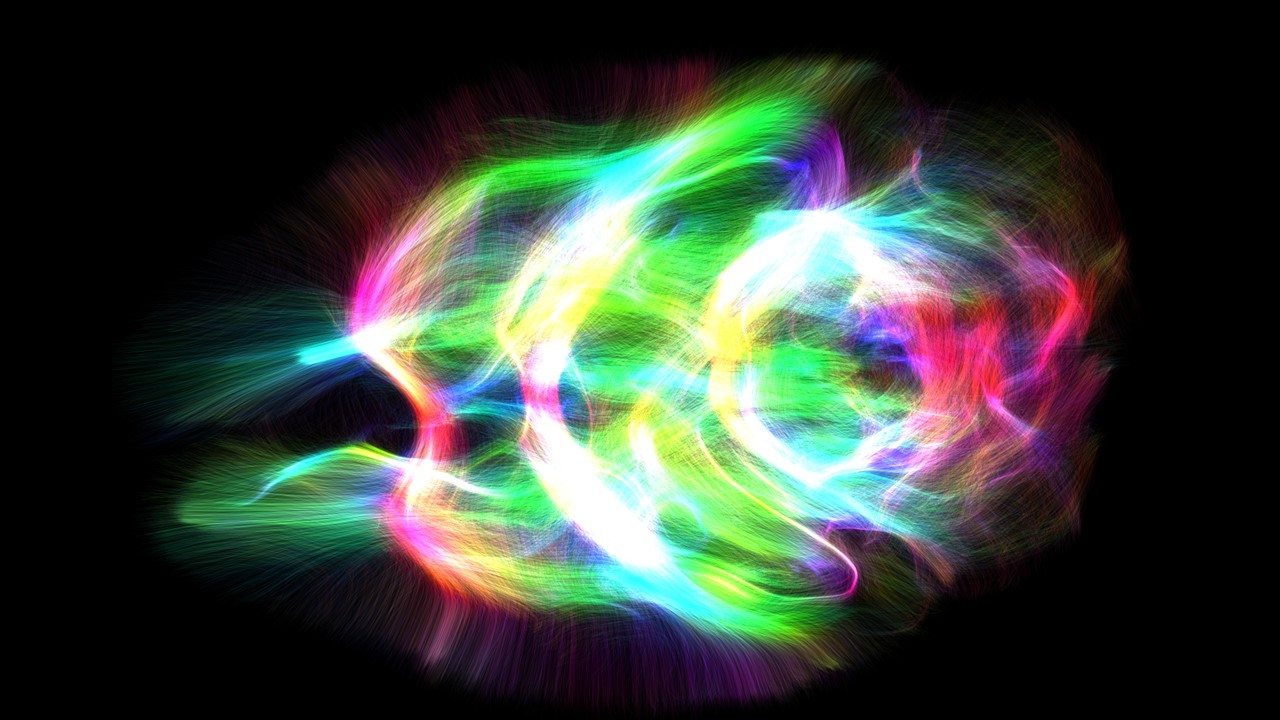The image features an abstract light pattern set against a pitch-black background. At the center, an intensely bright, dense cluster of light refracts and diffuses, creating a vivid display of intertwined colors including blues, greens, purples, oranges, reds, pinks, yellows, and whites. The central glow is vibrant and densely packed, resembling the effect of Neo markers scribbled tightly together. From this core, the light twists and bends, forming a coiled, fibrous, or wavy orb that appears almost three-dimensional. As the light radiates outward, it becomes finer and more dispersed, giving the appearance of fading into the dark surroundings. A subtle, blurry aura further enhances the ethereal and dynamic nature of the lighting. The overall aesthetic of the image is abstract, showcasing the captivating and intricate play of refracted light.